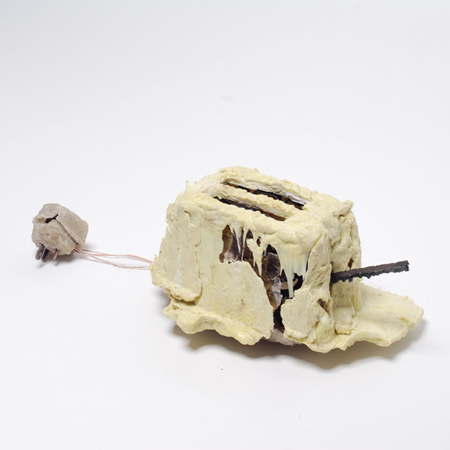The image depicts a toaster that is thoroughly covered in a thick, white clay-like substance that appears to be dripping down and enveloping the entire device. The background is a light gray, creating a stark contrast with the off-white material encasing the toaster. The appliance features a dark gray lever where a standard flat push-down mechanism would typically be. Both the toaster and its cord, which extends from the back and includes a three-prong plug, are covered in this clay-like substance, giving the objects an almost sculptural, artistic quality. Amidst the encasement, some dark sections are visible beneath the white material, hinting at the original toaster structure. The substance appears to be applied roughly, as there are visible cracks and uneven patches, particularly noticeable at the top and front of the toaster. A metal rod-like object protrudes from the lower right part of the scene, adding to the broken and deconstructed appearance of the overall setup. The image's neutral tones and the unrefined application of the material suggest an avant-garde or experimental art piece rather than a functional kitchen appliance.